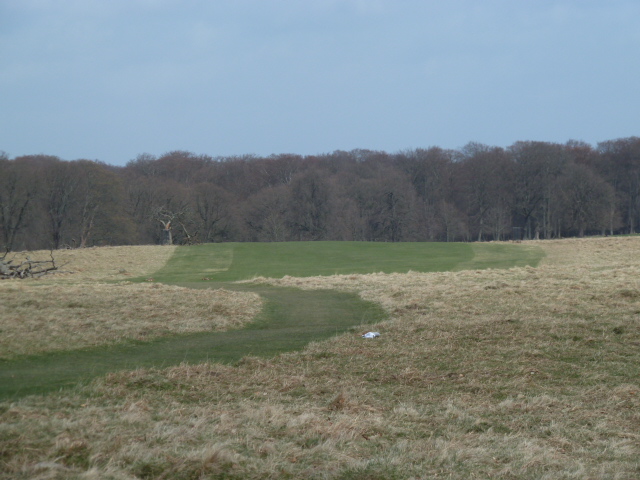This faded, out-of-focus color photograph captures an open field as seen outdoors during the day. The top third of the image is dominated by a clear blue sky, devoid of clouds. Stretching out below the sky in the far distance is a forest of bare, brown trees, indicating it might be fall or winter. The bottom half of the picture showcases a vast field divided into distinct sections. The center of the field features a greener, square patch of grass, suggesting it has been recently cut, surrounded by winding pathways. This green area is contrasted by the rest of the field, which consists of beige, dead grass on both the left and right sides. Towards the far left side of the image, there's a wood pile, adding to the rustic nature scene. The overall lighting is poor, and a small white object, possibly a bag or piece of trash, is slightly visible near the center of the image. There are no clear indications of the exact location or time period.